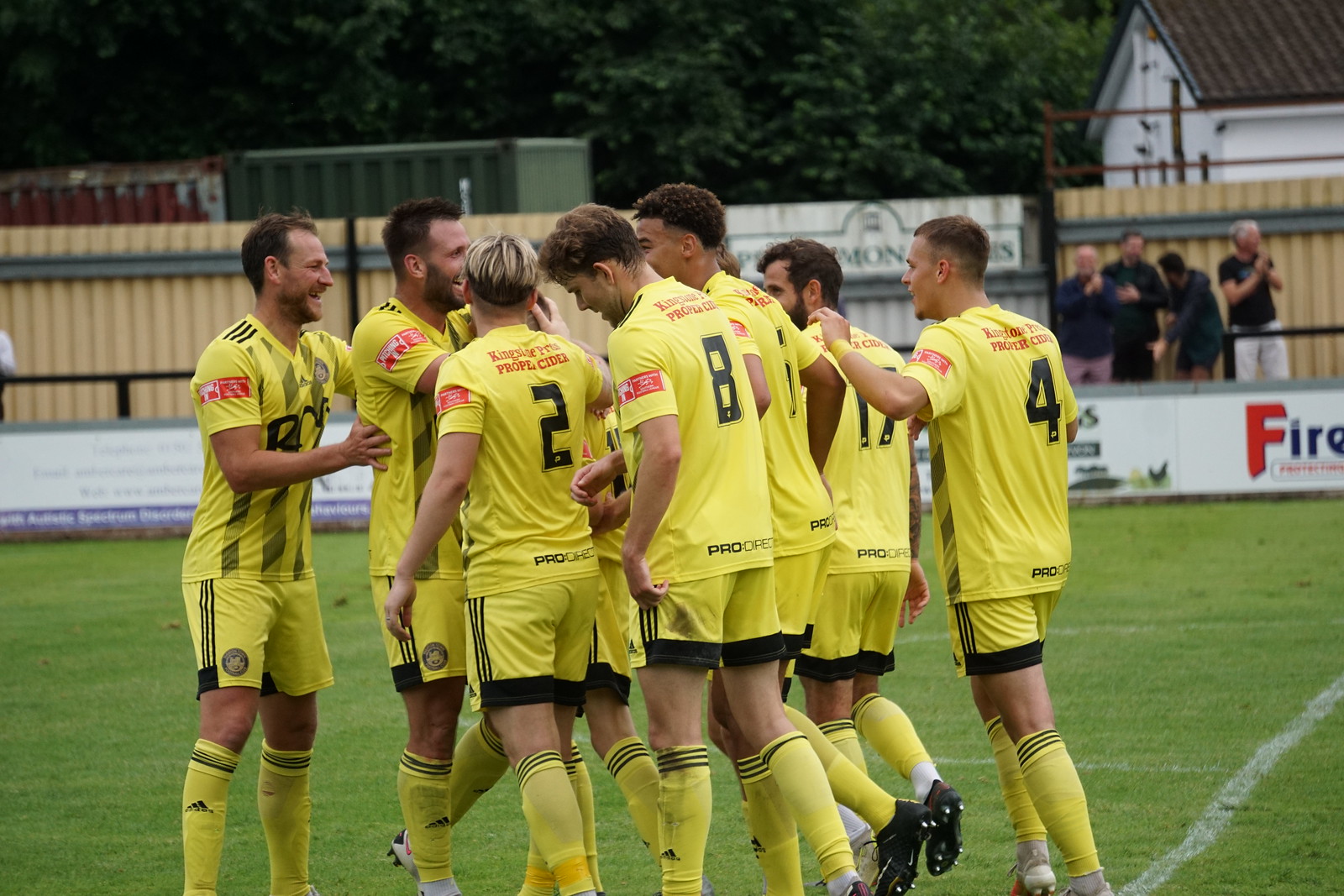This vibrant color photograph captures a team of seven male soccer players gathered on a lush green football field. They are all clad in bright yellow jerseys, shorts, and socks, which feature distinctive black stripes on the sides of their shorts and at the top of their socks. The scene seems to take place during a team huddle as the players, most of whom have dark hair except one with blonde hair, face each other with smiles. Visible on the backs of some players’ jerseys are the numbers 2, 8, 17, and 4, although some text on the jerseys remains partially obscured and unreadable due to wrinkles and angles. The backdrop includes green trees, parts of a house with a white facade and brown roof, and some metal storage containers or corrugated steel structures. Observing the team from behind a low metal rail and near a low wall adorned with advertisements are a few older men. The vibrant field further emphasizes the bright, lively atmosphere with its neatly painted white lines contrasting against the green grass.